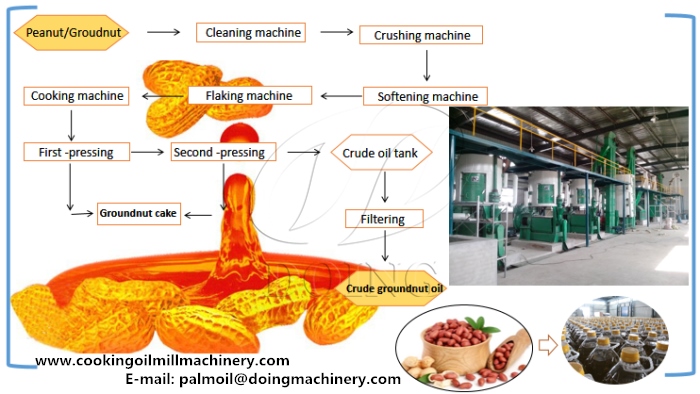The image is a detailed flow chart illustrating the process of transforming peanuts (or groundnuts) into crude groundnut oil, accompanied by a depiction of a peanut processing plant. The process begins with peanuts undergoing cleaning, followed by crushing, softening, flaking, and cooking. From there, the mush progresses to first pressing, which can either result in the creation of a groundnut cake or proceed to second pressing. After the second pressing, the output can again be a groundnut cake or it can continue to a crude oil tank. The final stages involve filtering, leading to the production of crude groundnut oil. The image also includes a depiction of the machinery used in each step of the process, with the entire chart outlined in blue lines on both the right and left sides. Peanuts in various forms, including shelled nuts and a bowl of peanuts, are visible. At the bottom of the image, there is a URL (www.cookingoilmillmachinery.com) and an email address (palmoil@doingmachinery.com), providing contact information for further inquiries.